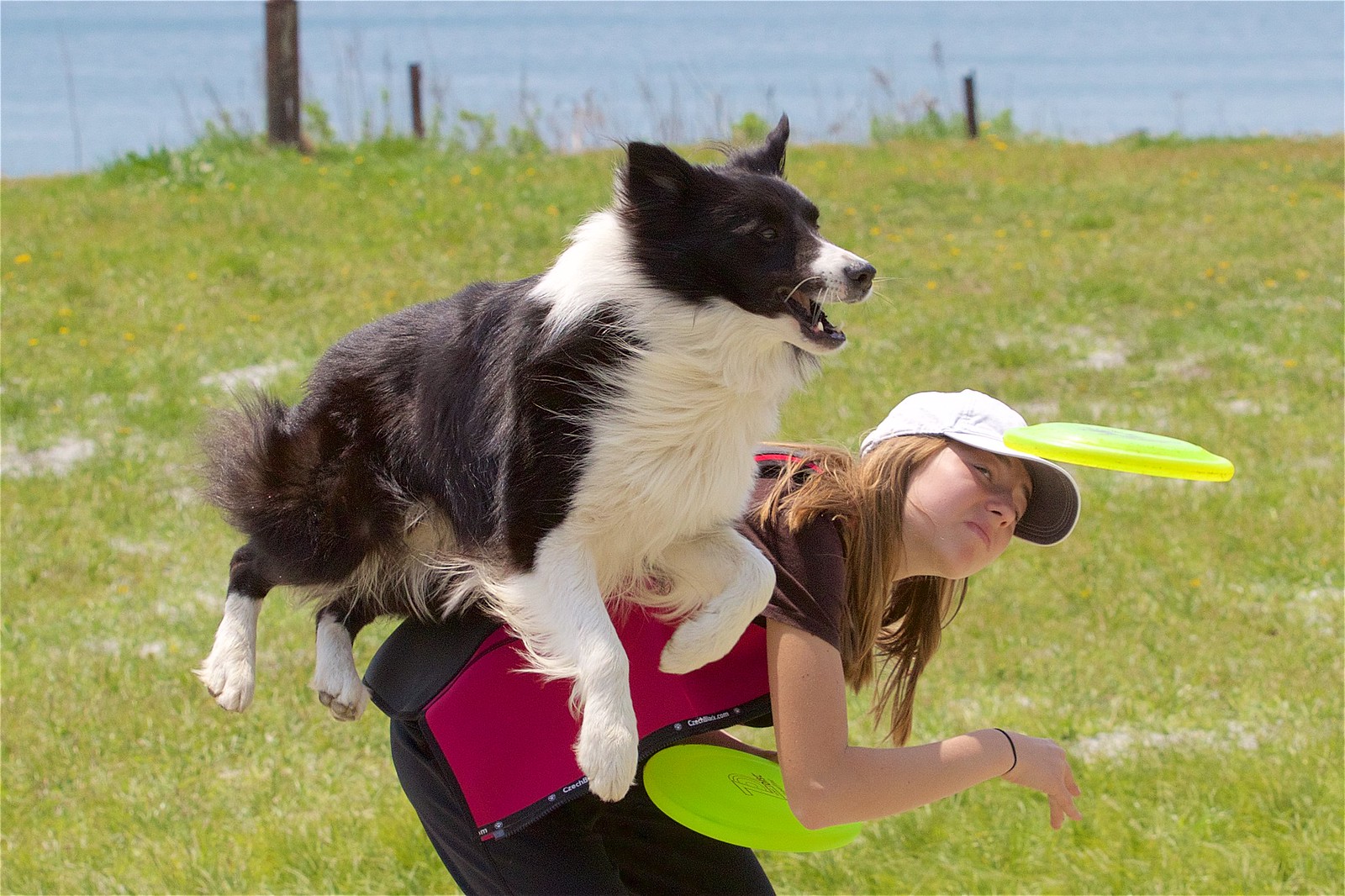In a vibrant, green meadow with wire fencing visible in the distance and a body of water on the horizon, a lively scene unfolds. A teenage girl with pale skin and long, fair hair, dressed in a red and black coat, black pants, and a white baseball cap, is kneeling down, seemingly to avoid an airborne dog. The girl holds a bright yellow frisbee in her left hand, having just thrown another, which is now the focus of a black and white border collie. The dog, with its eyes locked onto the frisbee and its mouth open in mid-leap, is soaring over the girl's back, its legs extended and its stomach possibly brushing against her. The energetic playfulness of the scene captures the bond between the girl and her agile dog, set against the scenic backdrop of lush grass and distant water.